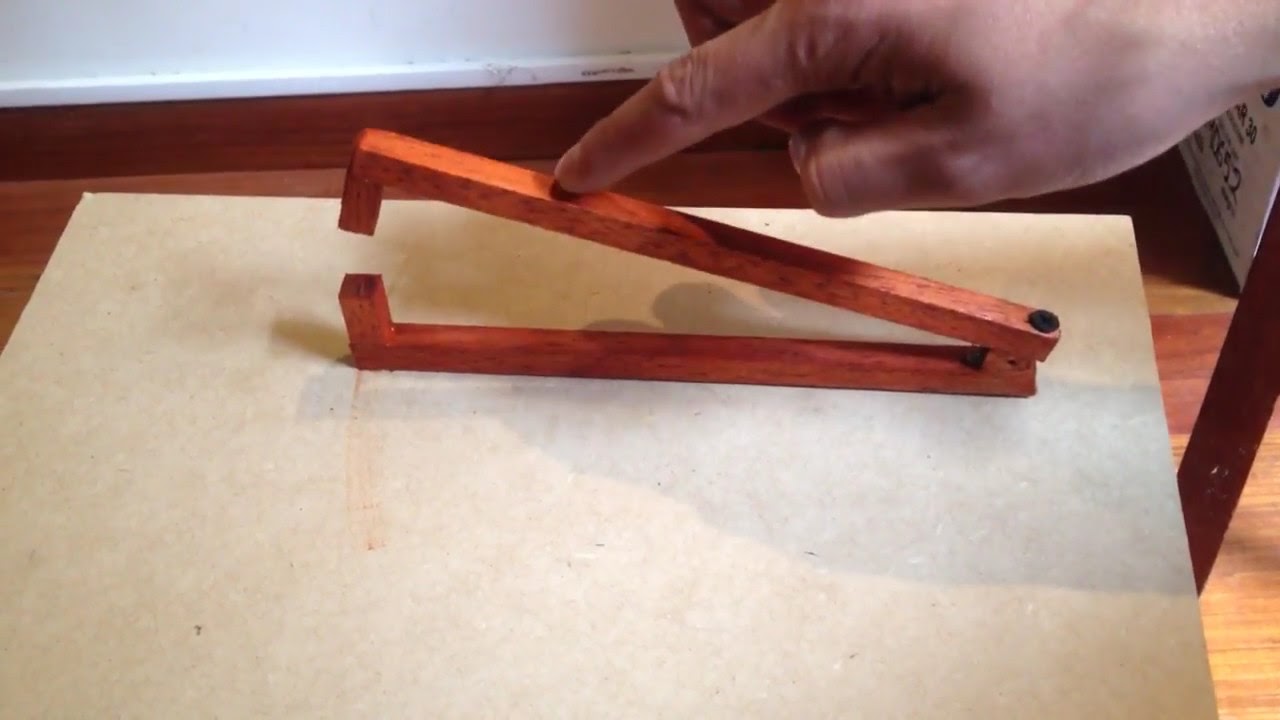In the image, a wooden mathematical tool resembling a compass is prominently featured at the center, surrounded by a variety of elements. The tool, crafted entirely from wood, stands upright and is being held by a hand entering the frame from the upper right corner. This hand, potentially belonging to a man, is positioned as if steadying or about to rotate the instrument. The tool rests upon a sheet of blue construction paper placed on a wooden surface, which might be a hardwood floor or tabletop. Additional items include a piece of white paper in the upper left and a box with indiscernible numbers in the upper right. The scene is set indoors, possibly within a workshop, illuminated by the warm tones of brown, white, off-white, tan, and black. The composition also reveals a subtle dust pattern around the tool, suggesting recent movement.